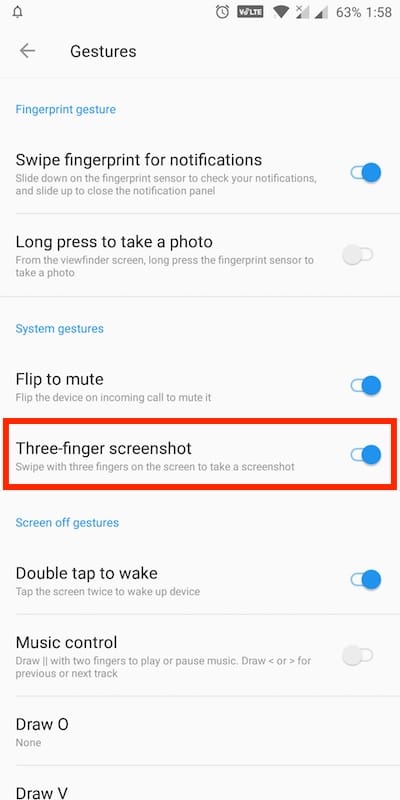A smartphone screen displays a detailed settings interface for gesture controls. At the top of the screen, indicators such as battery percentage, clock, and an alarm icon are visible. The primary focus is on the "Gestures" menu. A left arrow at the top of the menu suggests a way to exit this screen.

Below the "Gestures" header, there's a section labeled "Fingerprint Gestures" in smaller blue font. A description beneath explains that swiping the fingerprint sensor down opens the notification panel, while swiping up closes it. Additionally, a long press on the sensor can take a photo. This setting's slider button is currently enabled, indicated by being slid to the right.

The next section, "System Gestures" in bold blue text, lists three settings, all of which are turned on. These settings include "Flip to mute," "Three-finger screenshot" (highlighted with a red box), and "Screen off gestures." Under "Screen off gestures," options like "Double-tap to wake," which is enabled, allow users to wake the device by tapping the screen twice. The "Music control" option, described as using two vertical lines to play or pause, is currently turned off. Additionally, there are drawing commands such as "draw V" and "draw O," with corresponding functions highlighted in light gray.

The overall interface is designed with a clean, user-friendly layout, making it easy to toggle and understand various gesture-based controls for the smartphone.